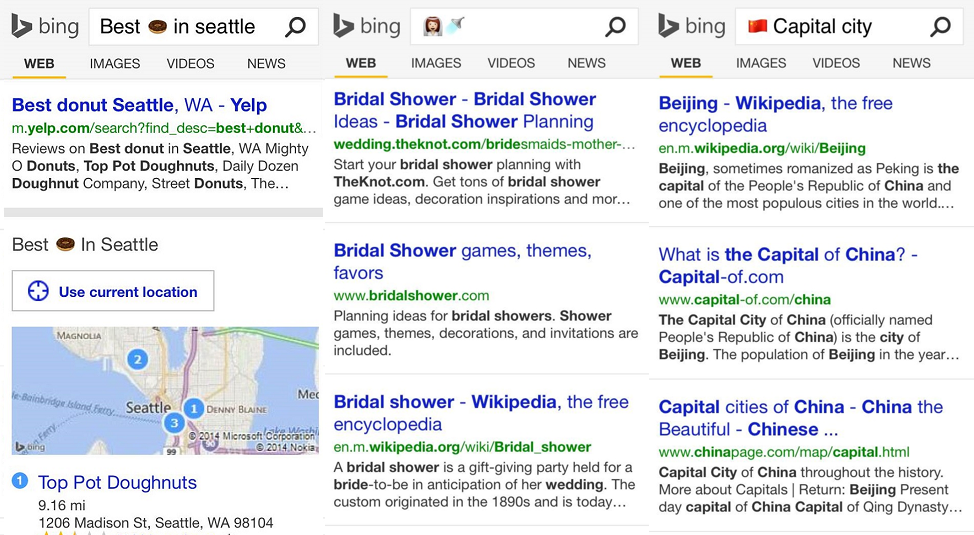The image displays search results for two different queries on a mobile device, spread across three pages. 

On the leftmost page, the first search result is highlighted in bold and blue text and reads: "Best donut Seattle". This is followed by "WA" in regular text, and then "- Yelp" in bold again. Beneath this bold text, there is a green link, which is part of the URL. Following this, a description appears: "Reviews on best donut in Seattle, WA Mighty O Donuts, Top Pot Donuts, Daily Dozen Donut Company, Street Donuts, etc." Below this description, there's a gray rectangular divider. 

Further down, there is a heading that reads: "Best 🍩 in Seattle". Next to this heading, there is a rectangular icon outlined in light gray, containing the text "Use current location" with a blue GPS signal icon to its left. 

A map is displayed beneath this, showing various highlighted areas marked with numbered bullet points indicating the locations of the donut shops.

On the second page, the search result is for "bridal shower". The title includes: "Bridal shower - bridal shower ideas - bridal shower planning". At the top, in the search bar, there are emojis of a bride and a shower to indicate the subject of the search. To the right, there's a flag, presumably of Beijing, with the text "Capital city". Below this, the result reads: "Beijing - Wikipedia, the free encyclopedia".

The third page lists search results related to the capital of China. The first title is "What is the capital of China - capital - of.com". The second title reads: "Capital cities of China - China the Beautiful - Chinese ...".